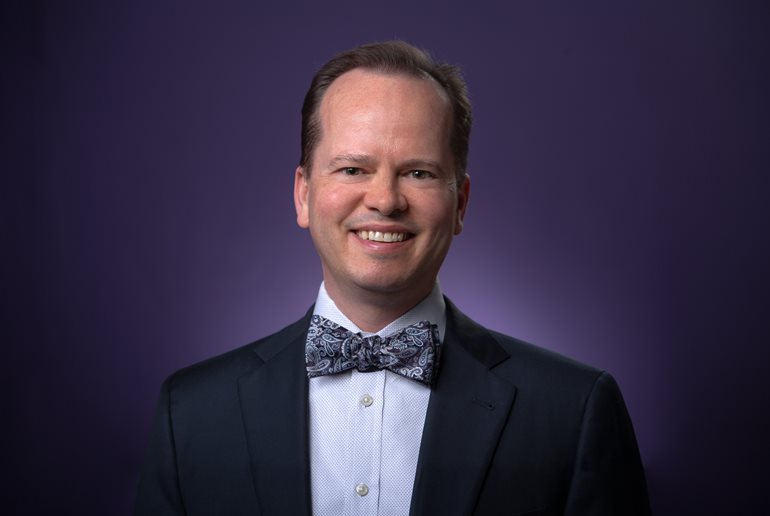The image features a white male standing against a purplish background with black edges. He is wearing a black suit jacket over a white dress shirt, and a distinctive large bow tie adorned with a slate-colored pattern featuring grays and whites. His hair, short and combed back, reveals a receding hairline and a prominent forehead. His eyes appear to be gray-greenish, and he is clean-shaven, showcasing a friendly smile that reveals his teeth. He has minimal eyebrows, a fairly large nose, and big ears. The headshot is centered on his upper body, mostly focusing on his cheerful face.